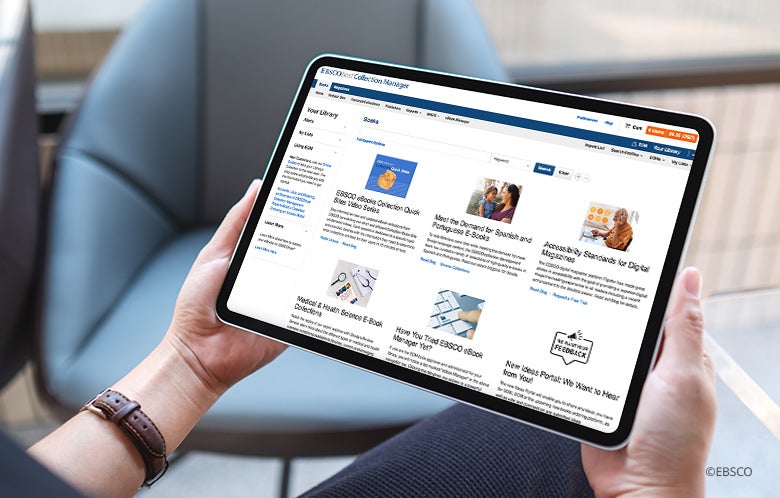The image depicts a person, whose gender is indeterminate, holding a tablet with both hands. The tablet, positioned towards the left of the photo, displays the EBSCO Collection Manager interface which includes various sections and articles. The background of the tablet screen is largely white, populated with different clickable content such as “EBSCO eBooks Collector Quick Video Series,” “Meet the Demand for Spanish and Portuguese eBooks,” “Accessibility Standards for Digital Magazines,” “New Ideas Portal Who Wants to Hear from You,” “Have You Tried EBSCO eBook Manager Yet,” and “Medical and Health Science eBook Collections.” Each section has images above and text below, although the images seem somewhat unrelated to the text.

The person’s thumbs are visible on either side of the tablet, with one hand extending from the lower left corner, showing part of the lower arm adorned with a leather watch band, and the other hand appearing in the lower right corner, cut off at the wrist. Part of their leg dressed in blue pants is also visible in the lower center of the image.

The setting includes a gray blurred chair in the background to the left of the tablet and a beige wall to the right. A copyright notice reading “© EBSCO” is located in the bottom right corner of the image.